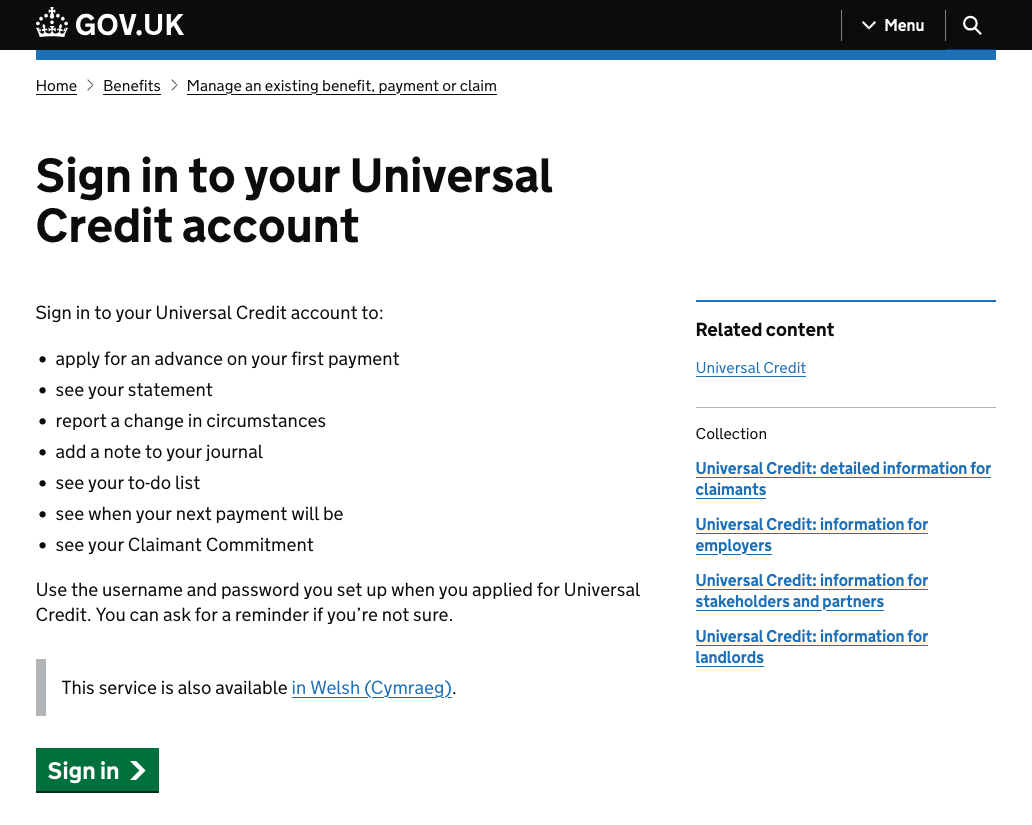The image depicts a webpage from the official gov.uk website, designed to provide support for those who are clinically extremely vulnerable to COVID-19. Prominently displayed in large, bold, black text is the message: "Get support if you're clinically extremely vulnerable to coronavirus." Beneath this statement is a green button labeled "Register/Update Your Details," indicating its function for users to update their medical status or register for assistance related to COVID-19.

The website features a cohesive, white background for a clean and straightforward presentation. At the top of the page, there's a distinctive black banner that hosts the gov.uk logo, accompanied by a thin blue stripe that runs horizontally. To the top right corner of this banner, a search field with a magnifying glass icon is available for user convenience.

Additionally, a blue "Related Content" link is present, presumably offering further resources or information related to the support available for vulnerable individuals. The design elements and layout clearly indicate that this is a part of the NHS's efforts to facilitate the updating and registration process for those affected by COVID-19.